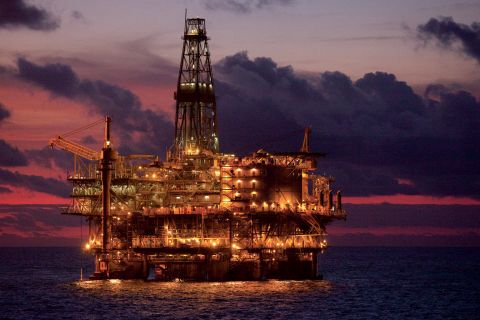The image captures a large, well-lit oil rig stationed in the middle of the dark ocean, with small waves rippling below it. The rig, a multi-storied mechanical structure, rises impressively from the water, appearing almost as if it is floating. A towering central assembly extends upward, nearly twice the height of the main structure itself, with a significant crane jutting off to the left. The photograph, taken at dusk, showcases a dramatic sky; dark clouds loom at the top while vibrant streaks of pink, orange, and red paint the horizon, suggesting a recent sunset. The mirrored lights from the rig shimmer across the murky blue ocean, highlighting the tranquil yet industrial setting.